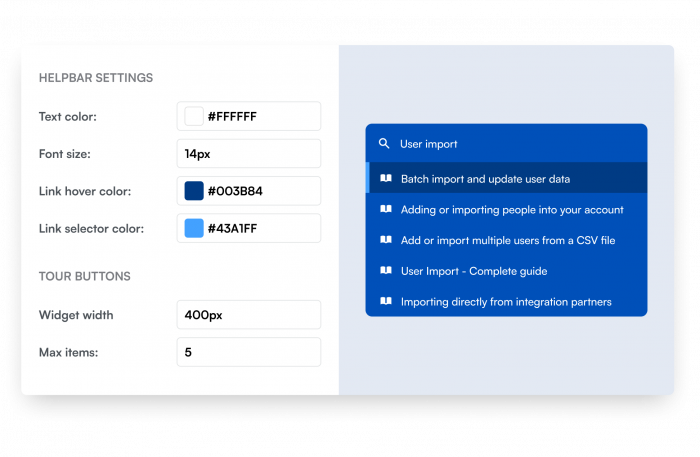**Descriptive Caption:**

The image depicts a user interface for configuring help bar settings, divided into two sections with distinct backgrounds. On the left side, against a white background, the upper left corner displays the title "Help Bar Settings" in a gray font. Below this title, several settings are listed:

- "Text Color" with a value of "#FFFFFF" (white),
- "Font Size" set to "14px",
- "Link Cover Color" indicated in a darker blue,
- "Link Selector Color" highlighted in a lighter blue,
- Below these options, a section labeled "Tour Buttons" is present with the following configurations:
  - "Widget Width" set to "400px",
  - "Max Times" specified as "5".

On the right side, set against a gray background, a pop-up window contains the title "User Import" with subsections detailing:
- "Batch Import - Update User Data": allowing the addition or importing of multiple users into an account,
- Instructions for adding or importing users from a CSV file.

This image provides a detailed and organized view of configurable settings for customizing the help bar and importing user data via a batch import process.